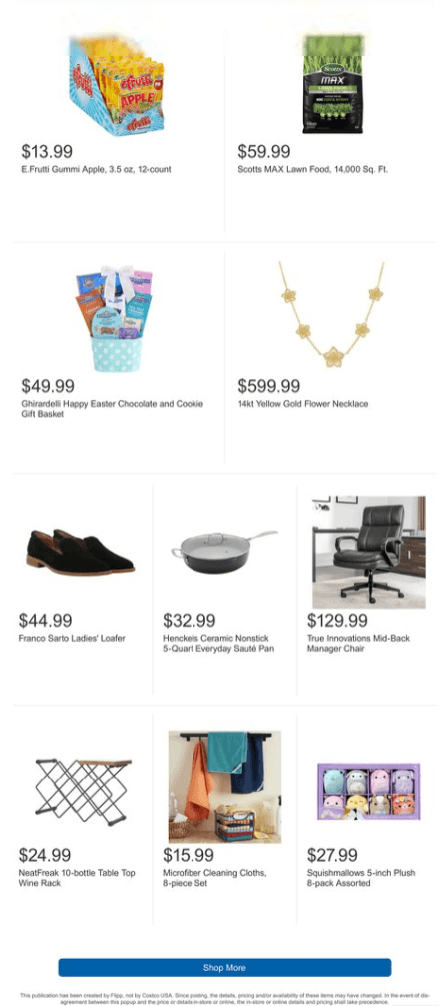The image is a screenshot from an online marketplace displaying various items for sale. At the top of the page, there's a brightly colored packaging of candy labeled "eFruit Guerrera's Apples," priced at $13.99 for a 12 count of 3.5-ounce packages. The packaging is orange with red writing. Below that, multiple items are arranged in a virtual storefront-like layout. 

Highlighted products include:
- A bag of lawn food priced at $59.99, featuring a black and green label with an image of grass.
- A "Ghirardelli Happy Easter Chocolate and Cookie Gift Basket" priced at $49.99, decorated in pastel colors with blue and white polka dots, as well as accents of purples, pinks, blues, and oranges.
- A 14 karat yellow gold flower necklace, which commands a price of $599.
- A pair of loafers available for $44.99.
- A ceramic nonstick pan listed at $32.99.
- An office chair priced at $129.99.

Each item is distinctively displayed with detailed visuals and clear pricing, set against the backdrop of the website's interface.